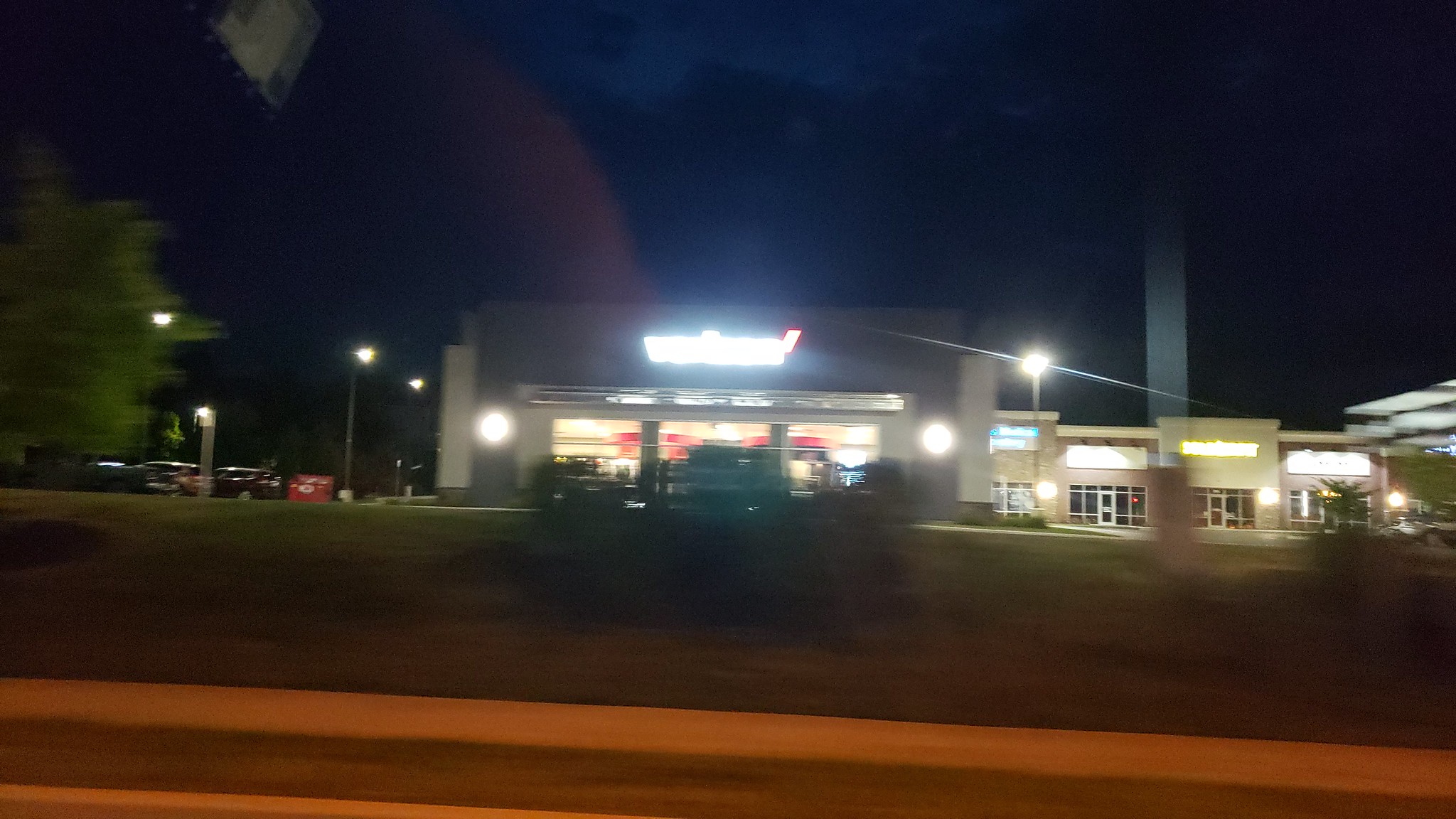The image captures an outdoor nighttime scene with a black sky as the backdrop. Central to the image is a brightly illuminated Verizon store, its sign glowing in vivid white and red lights. The photo is taken from the perspective of the road, featuring a sidewalk with a distinct white edge and a grassy dirt area adjacent to it in the foreground. 

To the far left, there is a parking lot filled with multiple cars, bordered by a row of trees and lit by several lampposts that cast a gentle glow over the area. On the right side of the image, multiple buildings with illuminated signs can be seen, their façades brightly lit against the dark sky. The overall scene is a juxtaposition of commercial vibrancy and the stillness of night, emphasizing the illuminated Verizon store as the focal point.